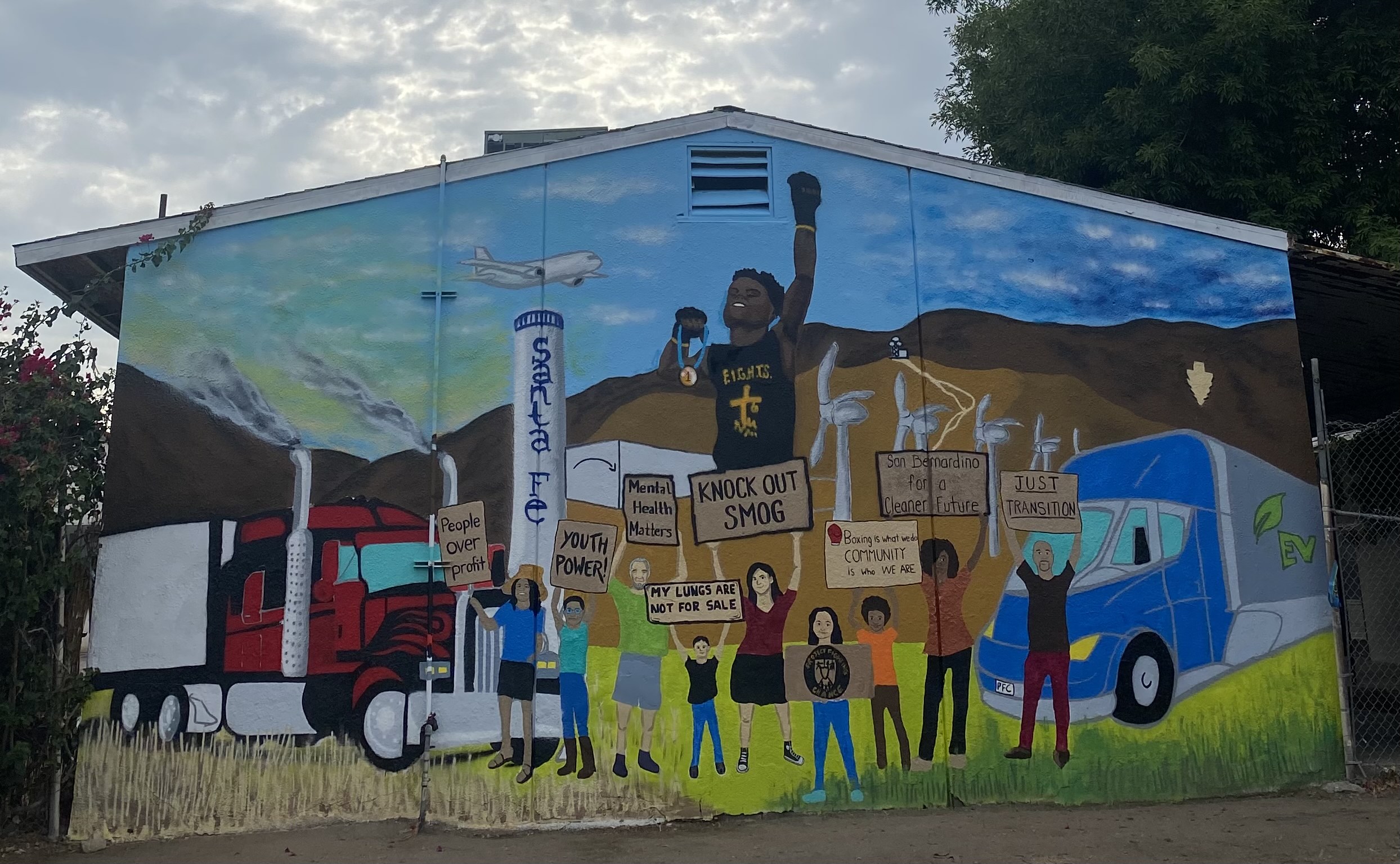The image is a detailed mural painted on the exterior of a building, possibly a two-story structure, which portrays a compelling narrative about environmental activism. At the forefront, there are two semi-trucks, one red on the bottom left and one blue on the far right, both emitting smoke. Between these trucks, a diverse group of children and adults hold signs advocating for environmental justice with messages like "Youth Power," "Knockout Smog," "Smog," "People Over Profit," "My Lungs Are Not For Sale," "Just Transition," and "San Bernardino for a Cleaner Future." Above the protesters, a large vent, slightly open, is noticeable in the middle of the image. A dynamic superhero figure, adorned with boxing gloves and holding a medal reminiscent of an Olympic award, leaps upward towards the sky, symbolizing the fight against pollution. The sky forms a serene backdrop with blue hues and white clouds, through which a passenger airplane soars. In the distance, wind turbines and a smokestack labeled "Santa Fe" are visible, indicating both the causes and potential solutions to smog. Surrounding the mural are trees, with a chain-link fence on the right and a ground covered in dirt, all under the gentle glow of sunlight breaking through the clouds.